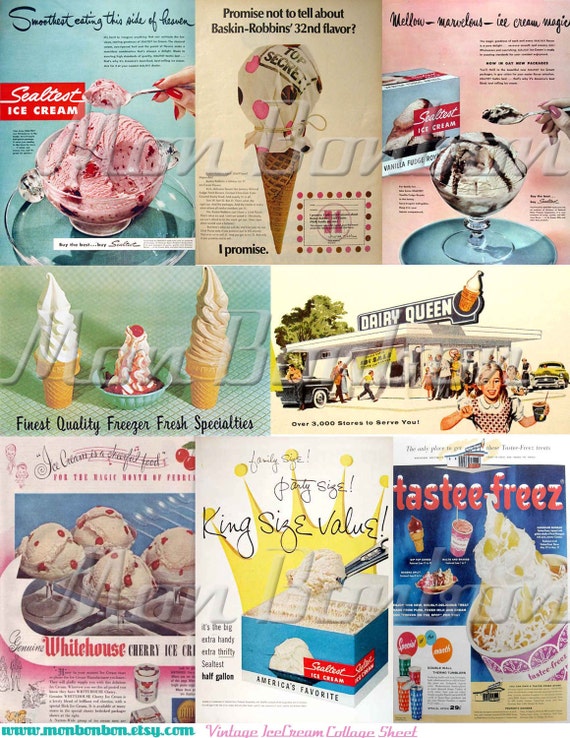This image is a vintage collage of eight ice cream ads from the 1950s and 60s. The ads are arranged in three sections: the top row features three smaller ads, followed by a middle section with two slightly larger ads, and then three more ads at the bottom. Prominently featured brands include Sealtest Ice Cream, Dairy Queen, Baskin-Robbins, Tasty Freeze, and White House Cherry Ice Cream. Sealtest appears three times, with one of their ads displaying strawberry ice cream in a bowl. Others show scoops of various flavors and ice cream servings in cake cones, sugar cones, and bowls. The designs are vibrant and colorful, with smooth, era-appropriate lettering. A faint watermark from www.monbonbon.etsy.com indicates this is a vintage ice cream collage sheet, available for purchase on Etsy.